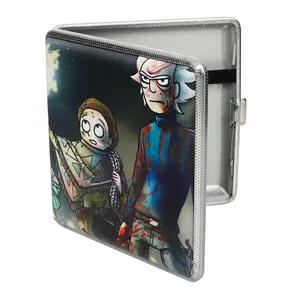The image depicts a compact, metallic-looking silver case, possibly plastic, resting against a pure white background. The case is slightly open, revealing a black strap inside and a clasp on the right side. The most striking feature is the detailed cartoon artwork on the front cover, visible only on the right side due to the partial opening. 

On the cover, to the right, stands a thin older man with spiky white hair and white eyes with black pupils. He is dressed in a long-sleeved blue shirt marred by red, rust-colored stains that cascade from the neck area downward, as well as a belt and pants that are visible down to his upper thighs. His expression is stern, and his right hand appears stained red. To his left is a smaller boy with short brown hair and wide eyes, looking up with a worried expression. The boy is draped in a blanket or scarf with a pinkish-bluish pattern, and he has a rope over his left shoulder. This careful design emphasizes both characters' striking features and the overall sense of a vivid narrative scene.